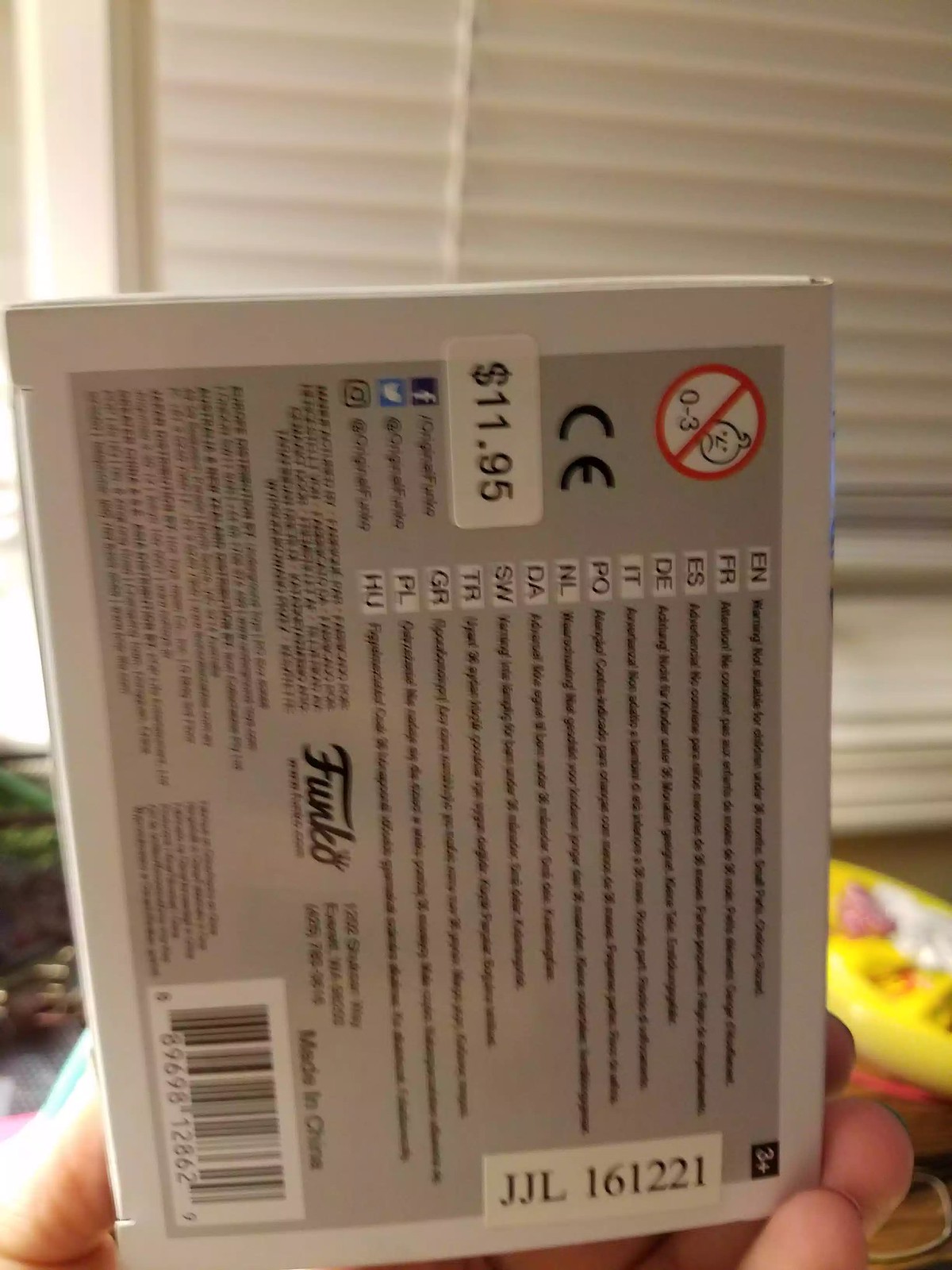In this photograph taken inside someone's house, a hand is holding up a white box with a gray panel featuring extensive multilingual text. The box, adorned with a price tag reading $11.95, also prominently displays a CE mark and a logo that spells out "Funko." An image at the top left features a red crossed-out baby symbol with the note "0-3," indicating it's not suitable for babies between zero and three years old. Below the barcode on the box are the words "Made in China." The background includes a window with white-painted frames and closed blinds, partially revealing what appears to be a baby in a yellow bed.